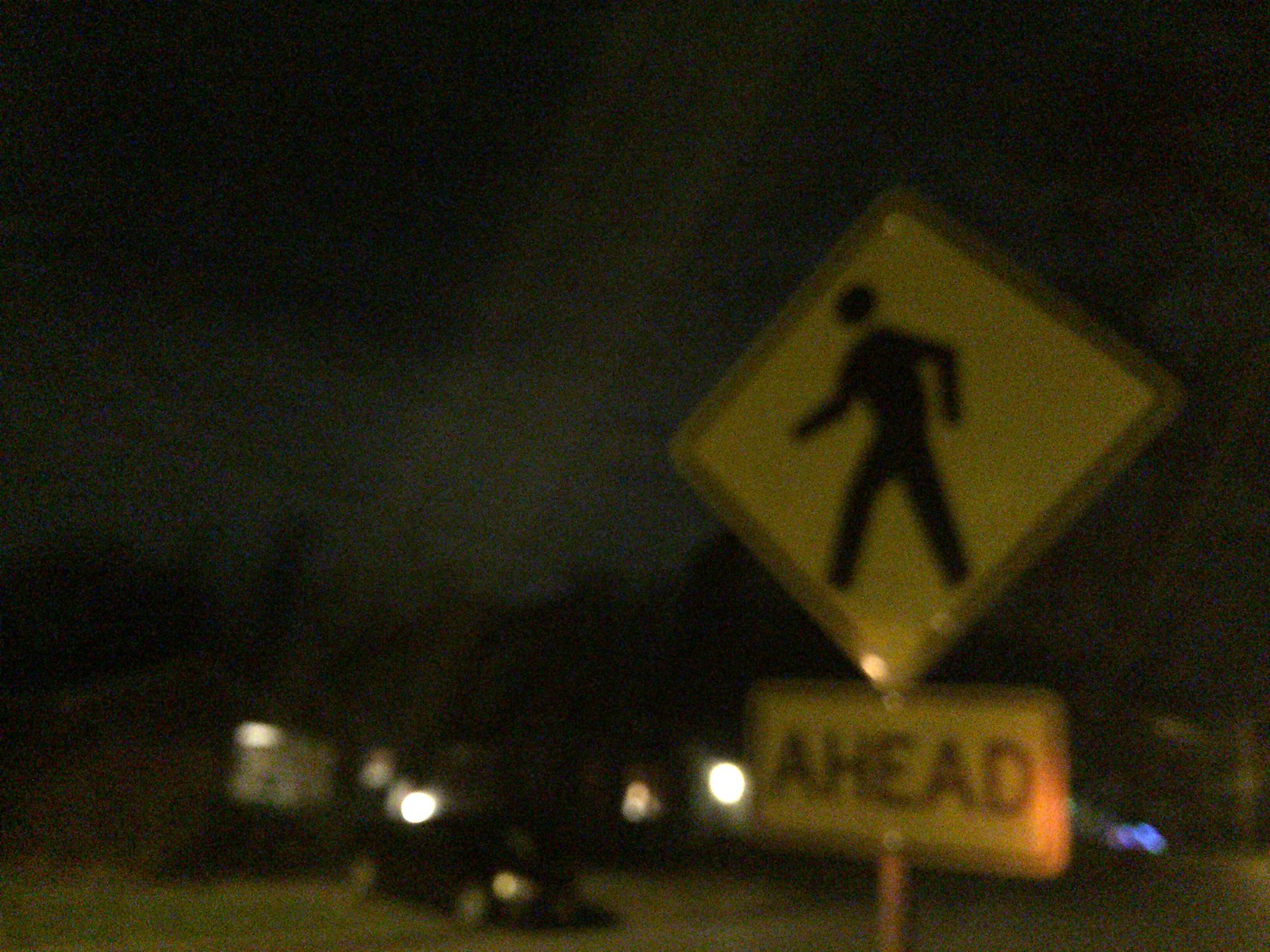This image depicts a street sign featuring a pedestrian icon set against a yellow background, with the word "AHEAD" written in bold black letters below. The sign serves as a warning to motorists that pedestrians may be walking or crossing ahead. In the background, one can see a residential street scene with a car parked in a driveway, various lights illuminating the area, and a small yard or grassy area. The sky is almost completely black, suggesting it is nighttime. The multitude of street lights further emphasizes the darkness of the evening. The main focus remains the cautionary pedestrian sign against the night backdrop.